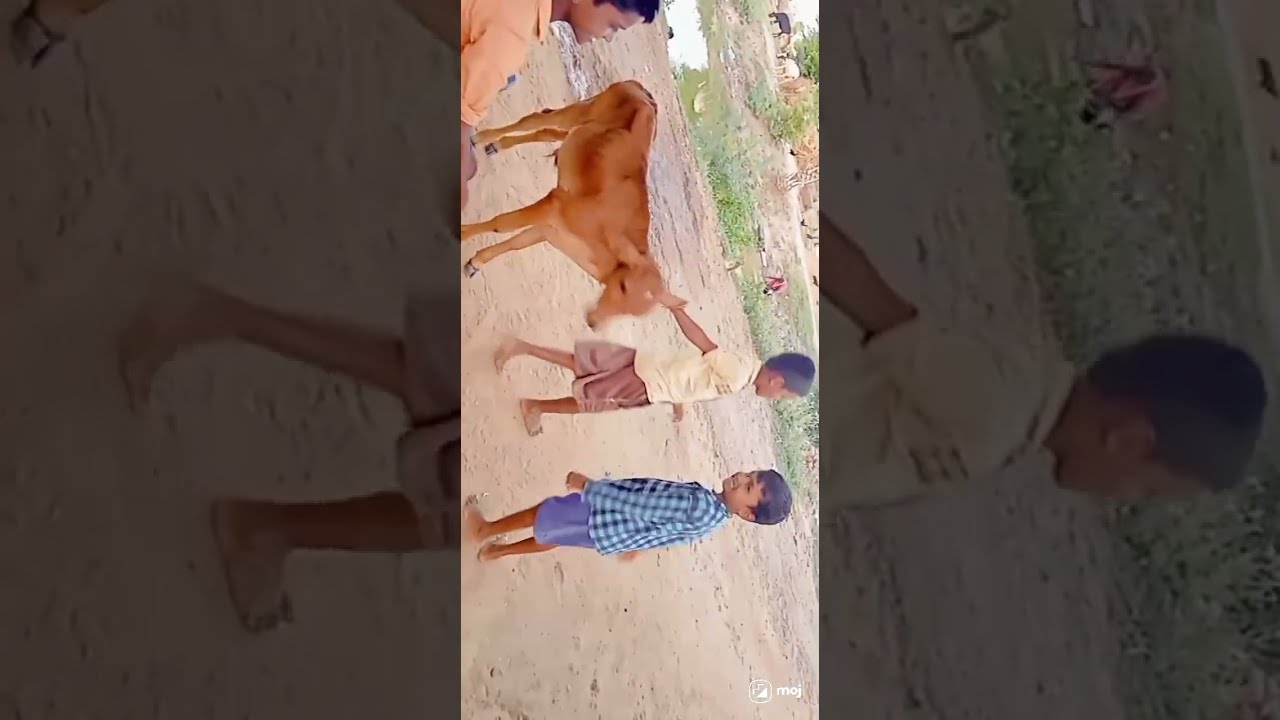The image is a screen grab from a video, viewed sideways, capturing a lively outdoor scene with three young Indian boys, appearing around ten years old. The boys, depicted on a dusty ground with occasional patches of grass, are seemingly engaged in playful activity with a baby cow. The central boy stands confidently in a yellow shirt and purple pants, gently guiding the reddish-brown calf by its ear, which appears calm and unbothered. Flanking him is another boy in a checkered blue shirt with matching blue shorts, while a third boy, partially off-screen in the top left corner, dons a light pink or orange shirt. The overall setting exudes a relaxed, playful atmosphere, with the distinct Moj watermark visible in the bottom right corner, adding to the narrative of children enjoying their time with their pet calf in a rustic, dirt-laden playground.